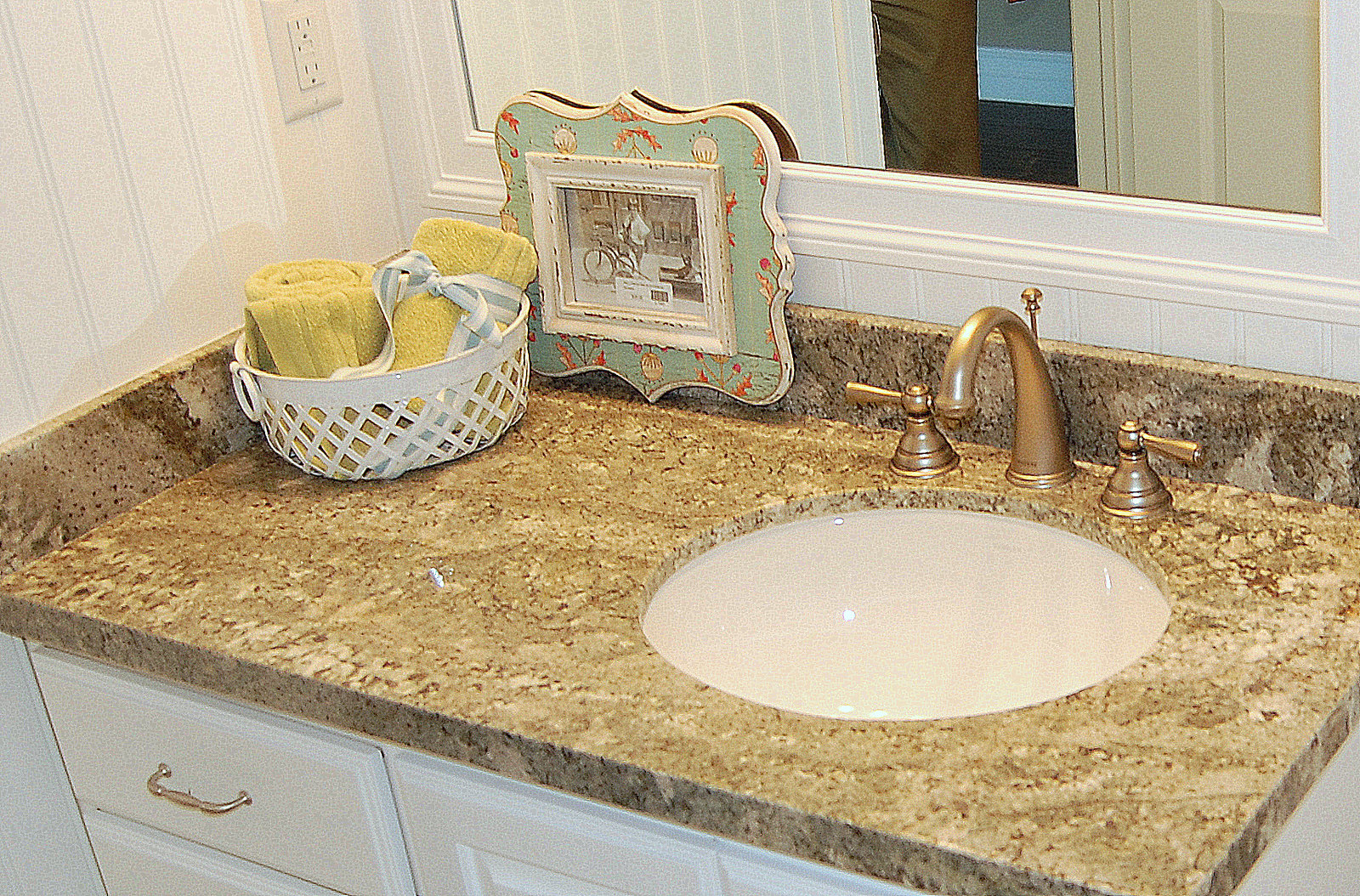In this image, we observe a meticulously arranged bathroom countertop. The centerpiece is a brass tap with accompanying handles, and behind it, a pull-top mechanism used to open or close the sink drain. The sink itself is a soothing cream color, set into a stunning light brown marble countertop that exhibits intricate white veining.

The wall behind the countertop is adorned with vertical white paneling, adding texture to the space. Embedded within this paneling is an off-white electrical fixture. Above the countertop hangs a mirror, bordered by a white frame with subtle ridging that echoes the wall's panel lines.

To the left, a white basket holds neatly rolled yellow towels, injecting a pop of color. Beside it, a framed black-and-white photograph depicts a person standing near a bicycle. The frame of this picture is bordered with layers of white, light green, red, and white again, with the outermost white layer decorated with bubble-like patterns.

Below the countertop, a white shelf is visible, equipped with a discreet silver handle. The mirror's reflection reveals an off-white door and a brown curtain, which likely conceals a bathtub. Additionally, a glimpse of gray flooring is seen at the bottom of the image, completing the bathroom's calm and cohesive design.